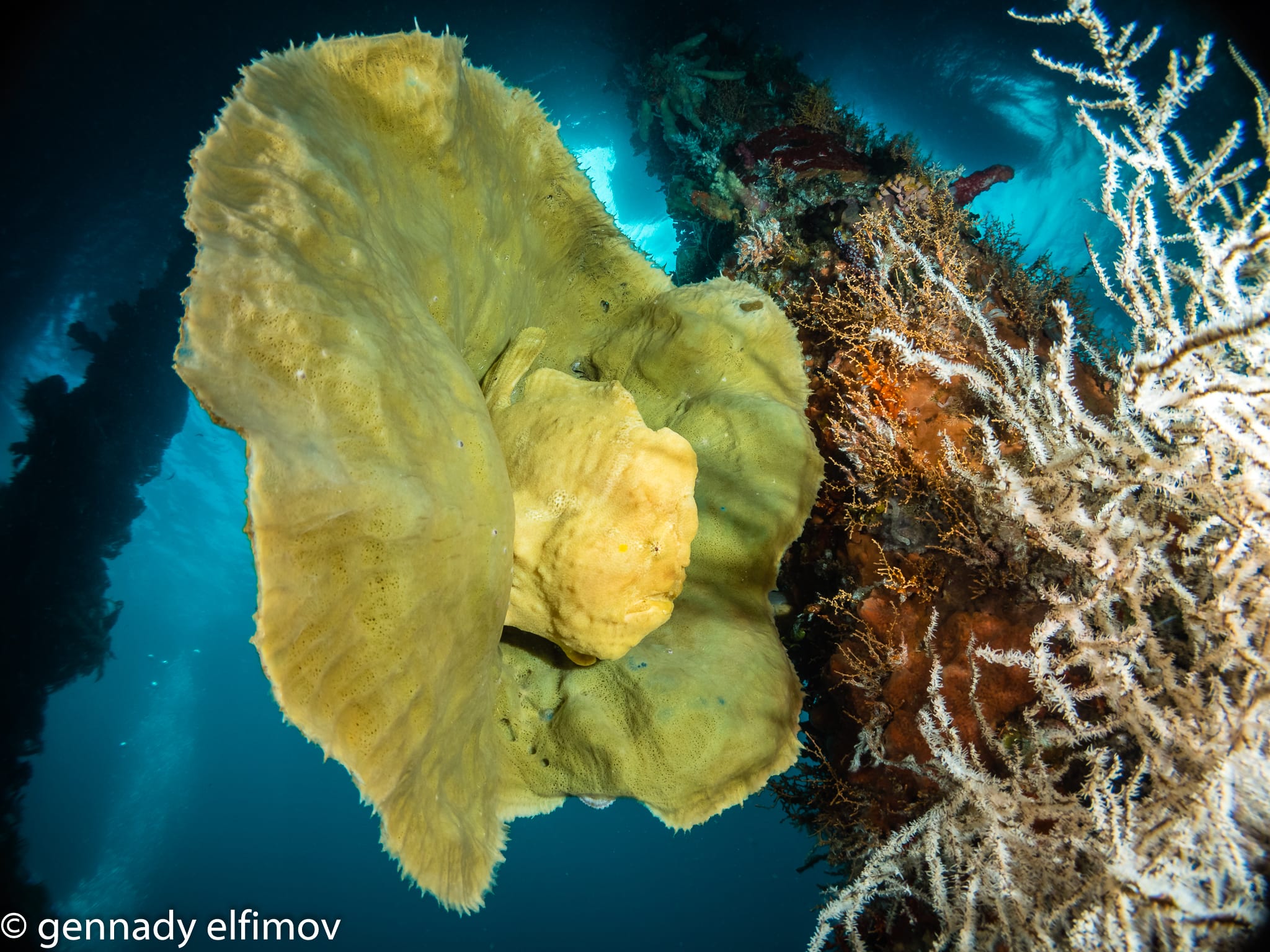An underwater photograph showcases a vibrant coral reef beneath the deep blue ocean. Dominating the center is a large yellow fish with a tail shaped remarkably like an oversized flower, accentuated with green and yellowish hues. Amidst the corals, the fish appears to be observing its surroundings, including a striking white and brown coral formation with thin branches on the right side of the image. Between the floral-like tail of the fish and the branching coral, there's a distinct brown triangular coral structure. The scene is captured with the backdrop of serene blue water, and in the bottom left corner of the image, it reads "Copyright Gennady Alfimov," indicating the photographer.